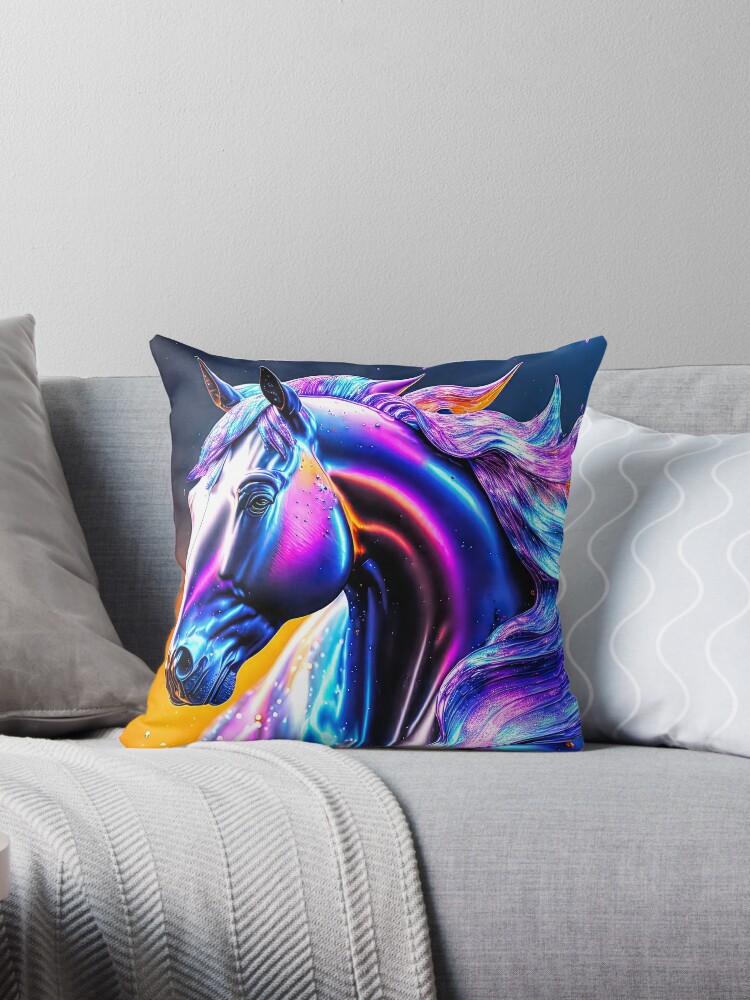The photograph captures a cozy, grey couch adorned with a few pillows and a blanket. Dominating the scene is a striking pillow at the center, showcasing a vibrantly colorful horse, with purples, blues, oranges, and pinks shimmering in an iridescent, metallic finish. This pillow stands out against its dark backdrop, drawing immediate attention. To the right of this eye-catching pillow is a white pillow featuring four squiggly white lines. A grey pillow is also slightly visible to the left, partially cropped out of the frame. The additional elements include a grey blanket draped over the couch, contributing to the overall comfortable and inviting atmosphere. The setting is complemented by a khaki-colored back wall, adding a neutral yet warm backdrop to the vivid and tranquil elements on the couch.